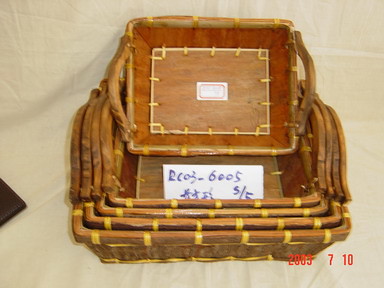This image, reminiscent of an old photograph, captures an elevated view of a stack of rectangular wooden picnic baskets with brown handles, arranged on a white towel or tablecloth. These baskets, characterized by their basket-weave bottoms and yellowish woven threads binding the wood, are nested within one another. The largest basket forms the base, with progressively smaller baskets nestled inside. The smallest basket is notably pushed slightly out, tipping on its side.

Prominently, a white piece of paper can be seen protruding from the center of the baskets, inscribed with the code "RC03-6005" and some Chinese characters. Additional markings include "S-5" in blue marker. At the bottom right corner, the numbers "2003-710" are visible, possibly indicating a timestamp of July 10, 2003. The overall background of the image is an off-white color, enhancing the rustic and slightly nostalgic feel of this scene.